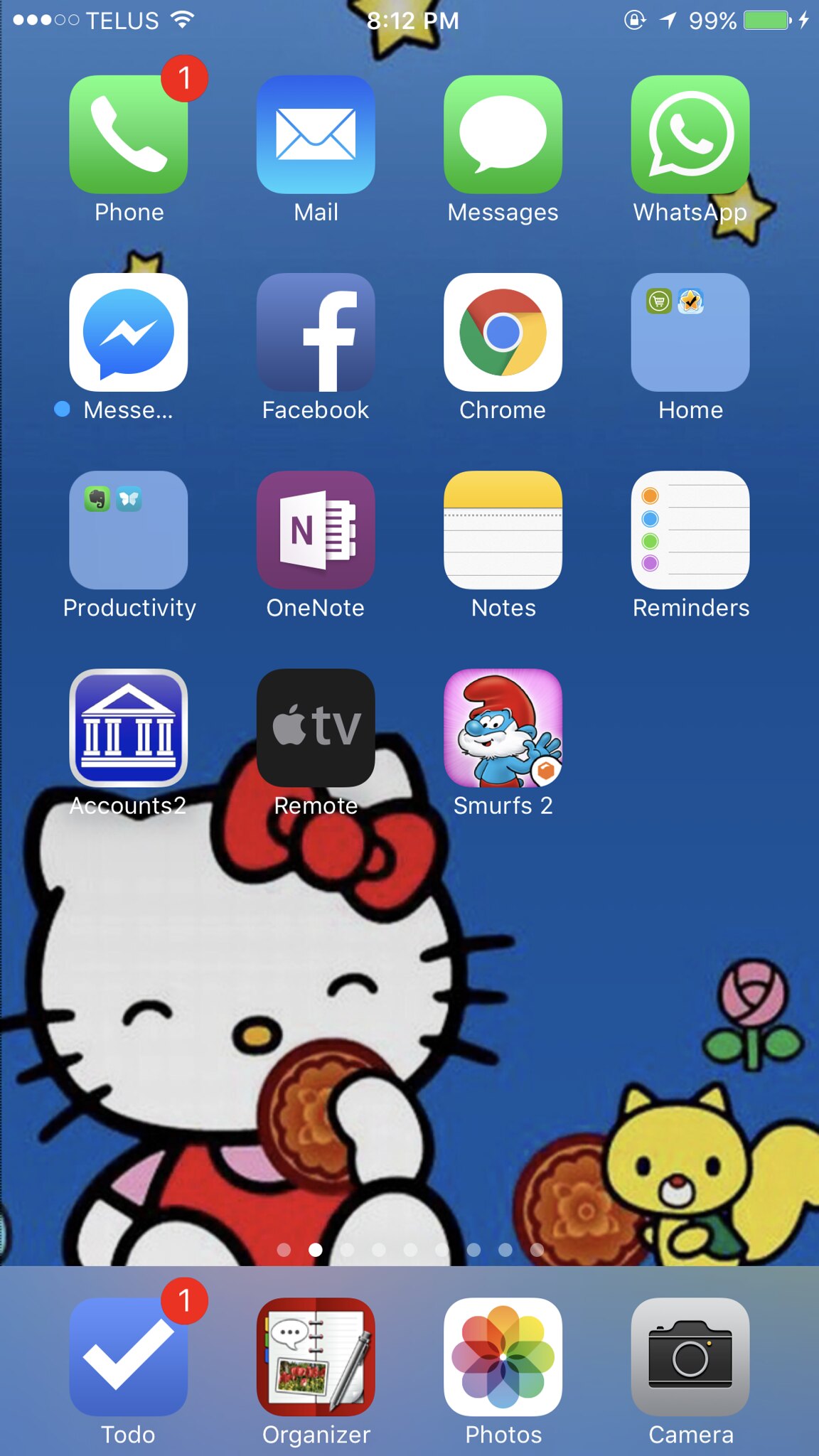A detailed screenshot of a smartphone screen is displayed, featuring a prominently placed illustration of Hello Kitty. Hello Kitty is depicted wearing a red jumper and a pink blouse, with her signature bow adorning her left ear. Her eyes are blissfully closed as she enjoys a tasty treat, demonstrating sheer delight. Beside her is a small yellow squirrel friend donning a green vest. Hello Kitty holds an intricately designed item, possibly food, while a little rose is also visible, adding a whimsical touch to the scene.

The phone screen itself has a blue background and displays a grid of 15 app icons. Notable apps include Apple TV, Smurfs, Facebook, Messenger, Phone, Mail, Messages, and WhatsApp, among others. There are also icons for a to-do list, an organizer, photos, and a camera. The layout appears relatively sparse compared to typical adult screens, hinting that it might belong to a child, although the presence of apps like Facebook causes some concern. This charming and organized layout captures a delightful and whimsical moment with Hello Kitty as the focal point.